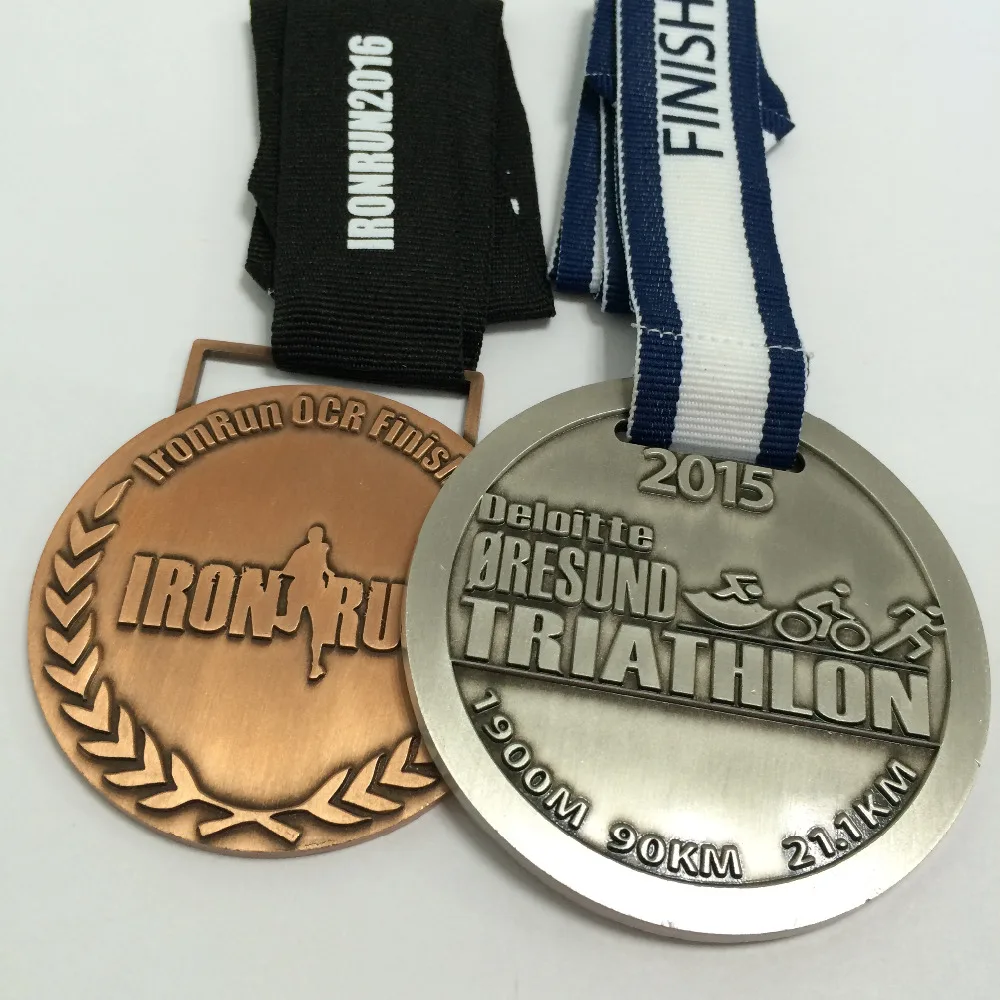The image shows two medals against an off-white background, each attached to distinct lanyards. The first medal, on the left, is bronze and labeled "Iron Run OCR Finish." It features a simplistic design with a logo of a running figure and is attached to a black strap with "Iron Run 2016" written in white letters, indicating the event year. The second medal, partially obscuring the first, is silver and associated with the Deloitte Horizonde Triathlon. This medal prominently displays "2015 Deloitte Horizonde Triathlon" along with icons representing swimming, biking, and running, denoting distances of 1900 meters, 90 kilometers, and 21.1 kilometers, respectively. It has a blue lanyard with a white stripe down the middle, featuring the word "FINISH" in blue letters.